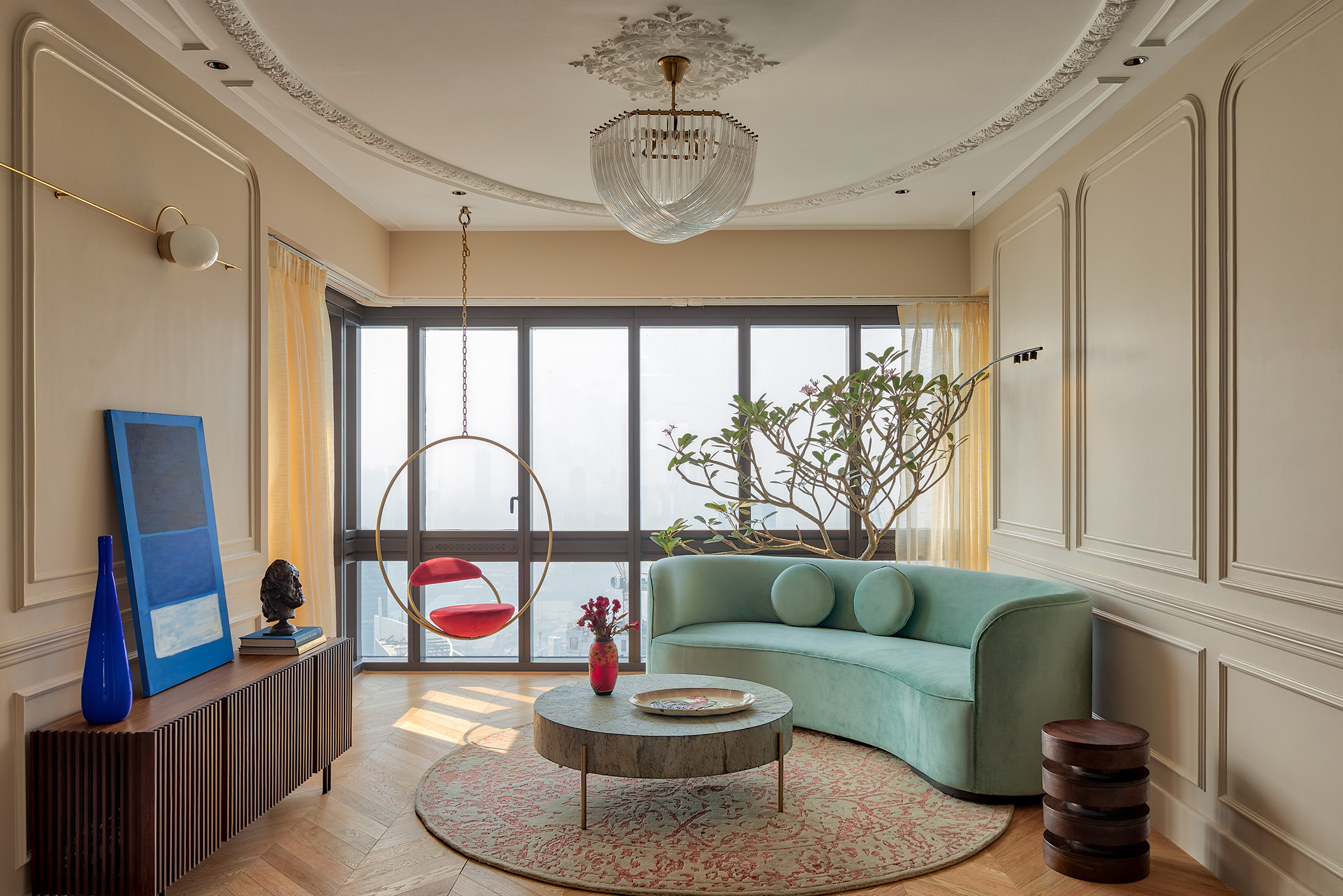In a luxurious, meticulously designed room with an air of wealth, the focal point is a magnificent chandelier hanging from a white ceiling adorned with intricate brocade detailing. The far wall is entirely made of windows, beautifully framed by white and yellow curtains that are drawn to the sides, allowing natural light to flood the space. Below the windows stands a striking tall bonsai tree, lending a touch of nature to the elegant setting.

To the left, a comfortable, light green velvet couch with rounded edges and two circular throw pillows invites relaxation. The couch sits atop a circular rug in tones of beige and rose, which rests on exquisite hardwood floors arranged in a herringbone pattern. In front of the couch is a round coffee table that features a colorful arrangement consisting of a red vase filled with vibrant flowers and a decorative plate.

Suspended from the ceiling by a gold chain on the right side of the room is a modern swing chair with a gold frame and plush red seat and back cushions, providing both a stylish and cozy seating option. Adjacent to the windows on the right is another large tree, resembling a ficus or an olive tree, enhancing the natural ambiance of the space.

On the left side stands an entertainment center or credenza, used for shelving and storage. Atop it sits a blue vase, a blue and white abstract artwork resembling a chalkboard, and a bronze bust accompanied by several books. The entire setting is carefully curated, with each element contributing to the room’s sophisticated and opulent aesthetic.